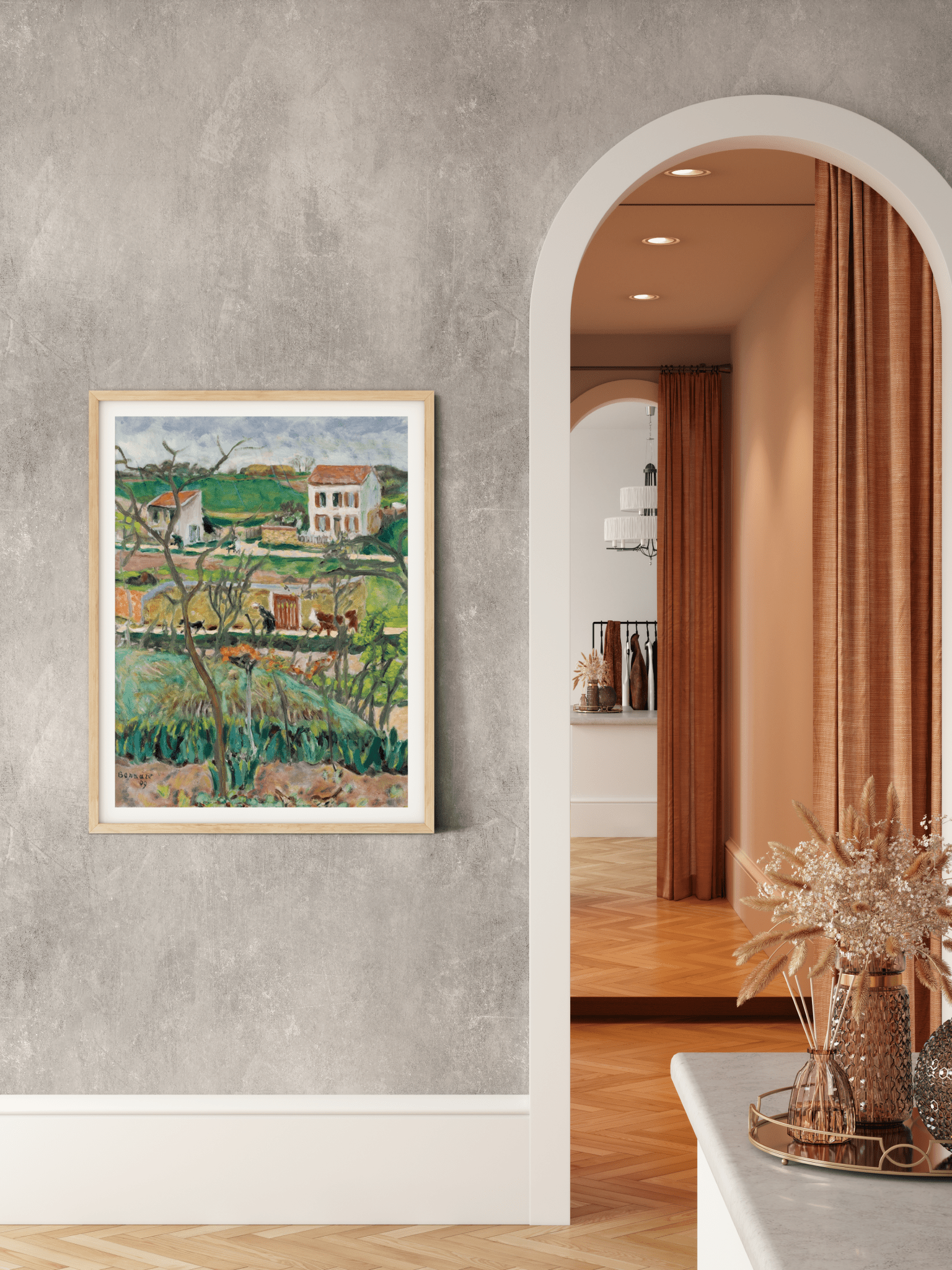The image captures a meticulously staged interior, prominently featuring a painting set within a brown wooden frame. This painting depicts a serene farmland scene with someone working the field, followed by a cow. In the background, there's a tall, two-story white house alongside a white shed, both adorned with red roofs. The painting is mounted on a gray painted wall, which contains a white archway on the right. Through this archway, one can see a tan-painted hallway with recessed round lighting on the ceiling and curtains used as doorways that are currently pulled open. The foreground houses a side table with a gray surface holding a reflective metal platter, an incense holder, a planter, and a floral arrangement of white and brown flowers. The entire area is unified by a wood parquet floor. Further back, a glimpse of a chandelier is visible, adding a touch of elegance to the scene. Additionally, one can observe baseboards, pink curtains, and a cluttered counter space in the far background, suggesting either the interior of a house or a store.